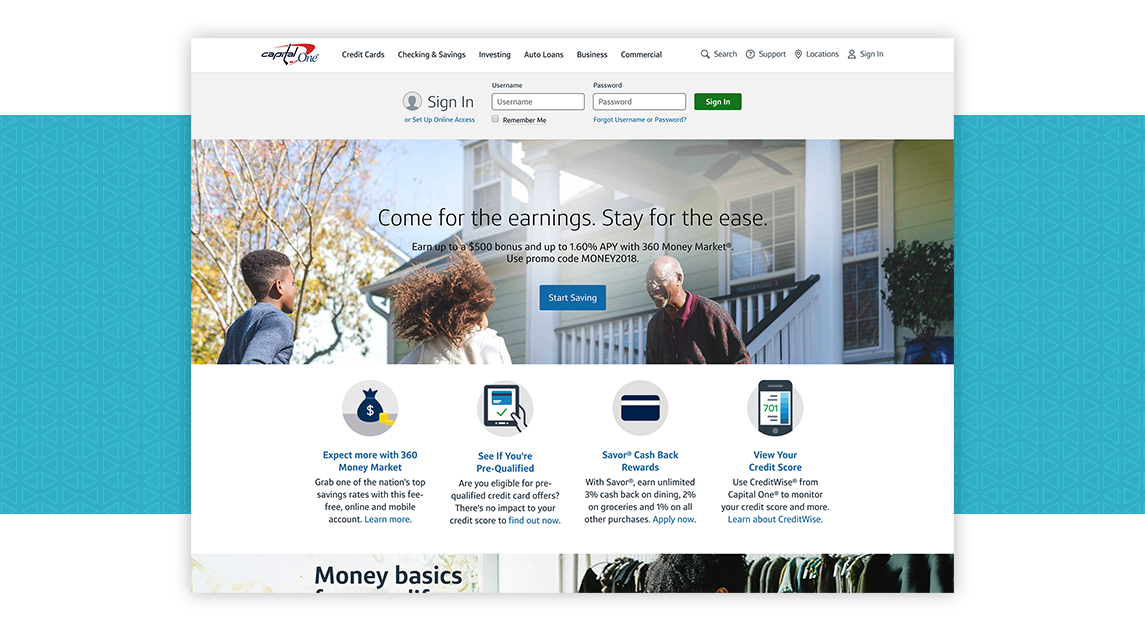The image features a vibrant background composed of various aqua-blue triangles pointing left and right. Overlaid on this geometric backdrop is the interface of Capital One's website. At the top left corner of the interface, the Capital One logo is prominently displayed, followed by a navigation menu that includes options for "Credit Cards," "Checking & Savings," "Investing," "Auto Loans," "Business," and "Commercial." Additional icons for search (magnifying glass), support (question mark), PIN management, location services, and sign-in (depicted with a person icon) are also visible.

Beneath the menu, a gray rectangular sign-in section is presented. It invites users to sign in or set up online access with fields for a username and password, a checkbox for "Remember Me," a link for forgotten login credentials, and a green "Sign In" button with white text.

Just below this section, there is an inviting promotional banner. It features a smiling older African-American gentleman, a young girl, and a young boy standing in front of a charming greenhouse with potted plants on the porch and a small set of stairs leading to the door. The accompanying text reads, "Come for the earnings, stay for the ease. Earn up to $500 bonus and up to 1.60% APY with 360 Money Market. Use promo code MONEY2018." A blue "Start Saving" button is also present.

The promotional content is followed by four icons, each enclosed in circles, representing various features and advantages of the 360 Money Market account:
1. A money bag icon labeled "Expect more with 360 Money Market" announces top saving rates and a fee-free online and mobile account, with a link to "Learn More."
2. An iPad icon labeled "See if you're pre-qualified" offers a no-impact credit check for pre-qualified credit card offers, with a clickable link to "Find Out Now."
3. A card icon labeled "Savor Cash Back Rewards" promotes earning unlimited cash back on dining, groceries, and other purchases, with an "Apply Now" link.
4. A phone icon with the number "701" on it labeled "View your credit score" encourages using CreditWise from Capital One for monitoring credit scores, with a link to "Learn about CreditWise."

The section concludes with the heading "Money Basics," although the content below is cut off and not visible in the image.